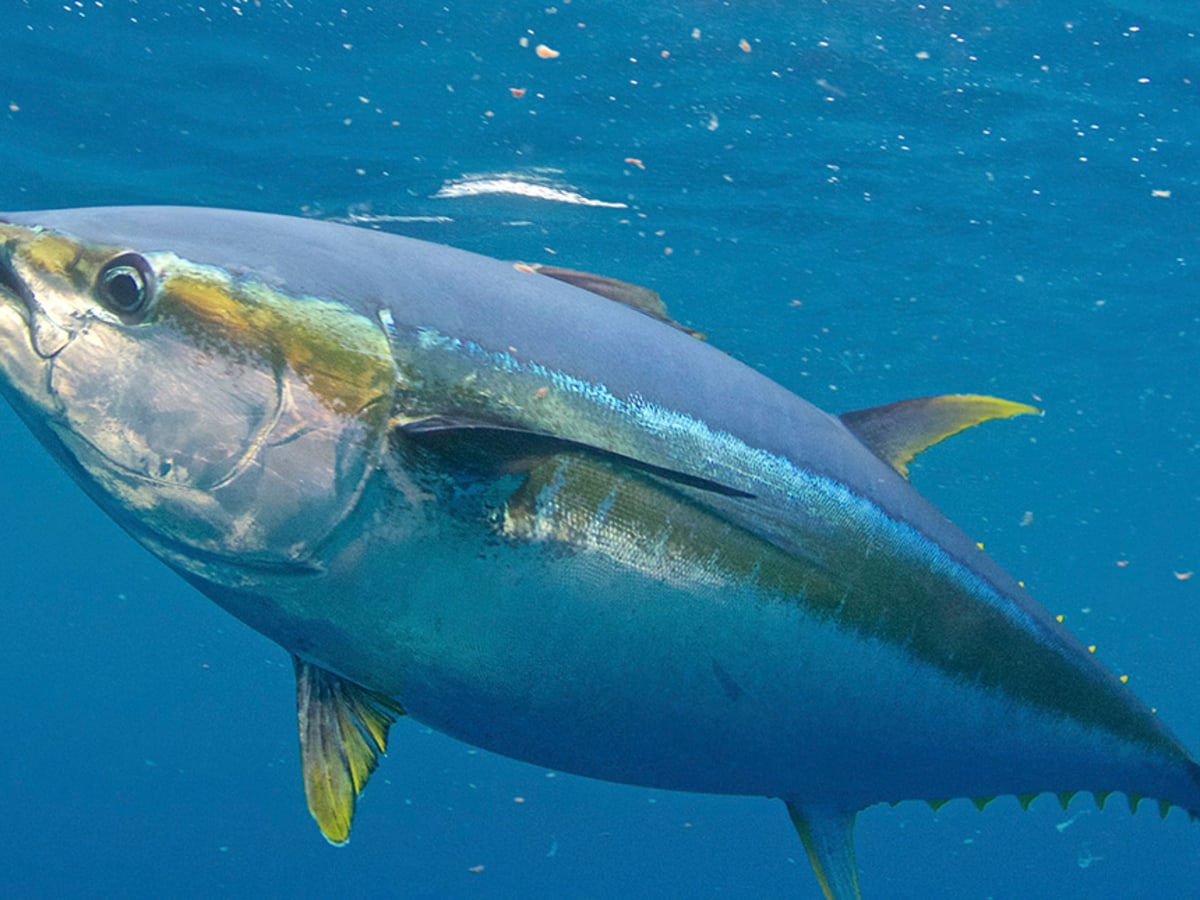The image captures a close-up view of a large, reflective silver fish swimming underwater in light blue, clear water with floating particulates, resembling fish food. The fish's body spans nearly the entire frame, with its mouth partially cut out on the left and the tail on the right. It has a detailed physique, featuring black eyes with blue backgrounds, lines and ridges around the gill area, and a sharp-edged dorsal fin. The scales and underside of the fish exhibit a scaly texture with hues of yellow, green, and gray. A yellow streak runs from its eye towards the side fin. Along the bottom, past the lower fin, the fish shows yellow spikes, giving it a distinct and colorful appearance. The reflection of a white line from above is visible in the water, adding to the scene's depth. The detailed markings and unique features suggest the fish could be a tarpon, although this identification is not certain.